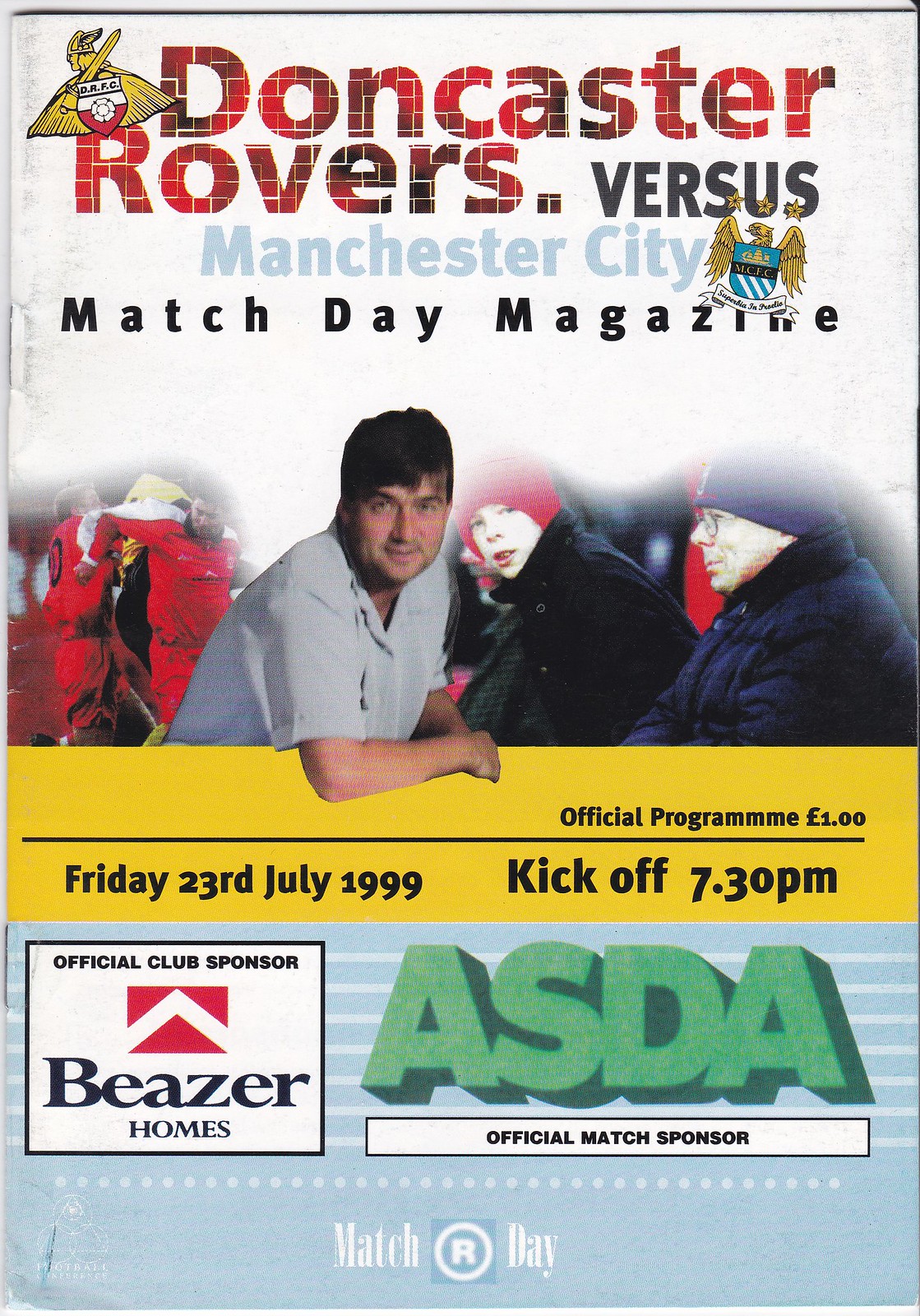The image features an old and slightly faded match day program booklet for the Doncaster Rovers versus Manchester City game, dated Friday, July 23, 1999, with a kickoff at 7:30 p.m. The cover is white with the text "Doncaster Rovers" in red and "versus Manchester City" in lighter blue, followed by "Match Day Magazine" in black. The booklet is bound by two staples and priced at one pound.

The top left corner showcases a yellow Viking holding a sword and a red and white shield with a soccer ball. On the bottom right next to "Manchester City" is a gold eagle and a shield in blue, gold, and white stripes with a ribbon beneath it in black text.

Centrally, there's a photograph of people, possibly including the coach, players, and children, all dressed warmly in red and black coats with snow hats, indicating cold weather. The exception is a man in a short-sleeve dress shirt in the front, leaning over a yellow bar running across the image. The left side features individuals in white and red jerseys and pants.

Under the photograph, a black line separates the text "Official Program £1" and the match details. Additionally, in a box on the left side, the bottom part of the graphic includes "Official Club Sponsor Beezer Homes" in black, while to the right of that, "ASDA," the official match sponsor, is displayed in green.